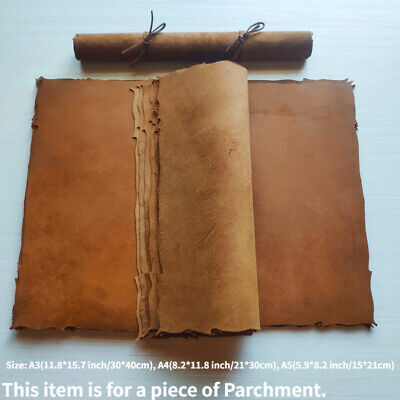The photograph showcases a piece of antique-looking parchment lying on a white surface. The parchment appears to be made of animal skin, featuring a range of brown hues from honey-colored to deep brown. This parchment is notably unused, with blank pages that have jagged, unprofessional edges as if they were torn rather than neatly cut. In the center of the piece, several pages are flipped, displaying their untouched nature. Above this parchment, there is a rolled-up scroll elegantly tied with two pairs of small ropes or twine. The backdrop, although predominantly white, has a light blue tint. At the bottom of the image, text details the item as "for a piece of parchment" and specifies the available sizes—A3, A4, and A5—along with their dimensions both in inches and centimeters. The photograph might be intended for a product listing, indicating that the parchment is for sale as individual sheets, possibly for crafting personalized journals, mementos, or special keepsakes like wedding vows.